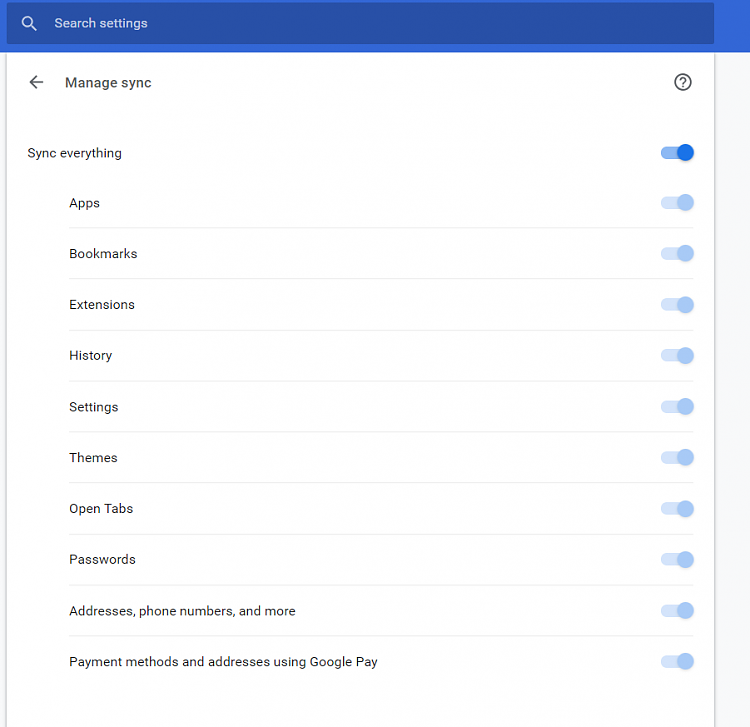This is a screenshot of a settings page, likely from an app or a browser. At the top, there is a blue header containing a darker blue search box with the label "Search settings" in white font. Below this header, the main content area has a white background displaying various options.

The top section is titled "Manage Sync," and to the left of this title, there is a back arrow for navigating to other options. To the far right of the title, there is a circular icon with a question mark inside, indicating help or additional information.

The first visible option under "Manage Sync" is the "Sync everything" toggle switch. This toggle is turned on, indicated by its highlighted blue color, which is more vivid compared to other options. Because the "Sync everything" option is enabled, additional syncing options are active. These include:

- Apps
- Bookmarks
- Extensions
- History
- Settings
- Themes
- Open tabs
- Passwords
- Addresses
- Phone numbers
- Payment methods and addresses using Google Pay

Given the mention of Google Pay, this settings page is likely associated with the Google Chrome browser or a related Google service. The overall background of the screenshot has a slightly grayish-white tint, but the detailed settings area is prominently displayed on a white background.